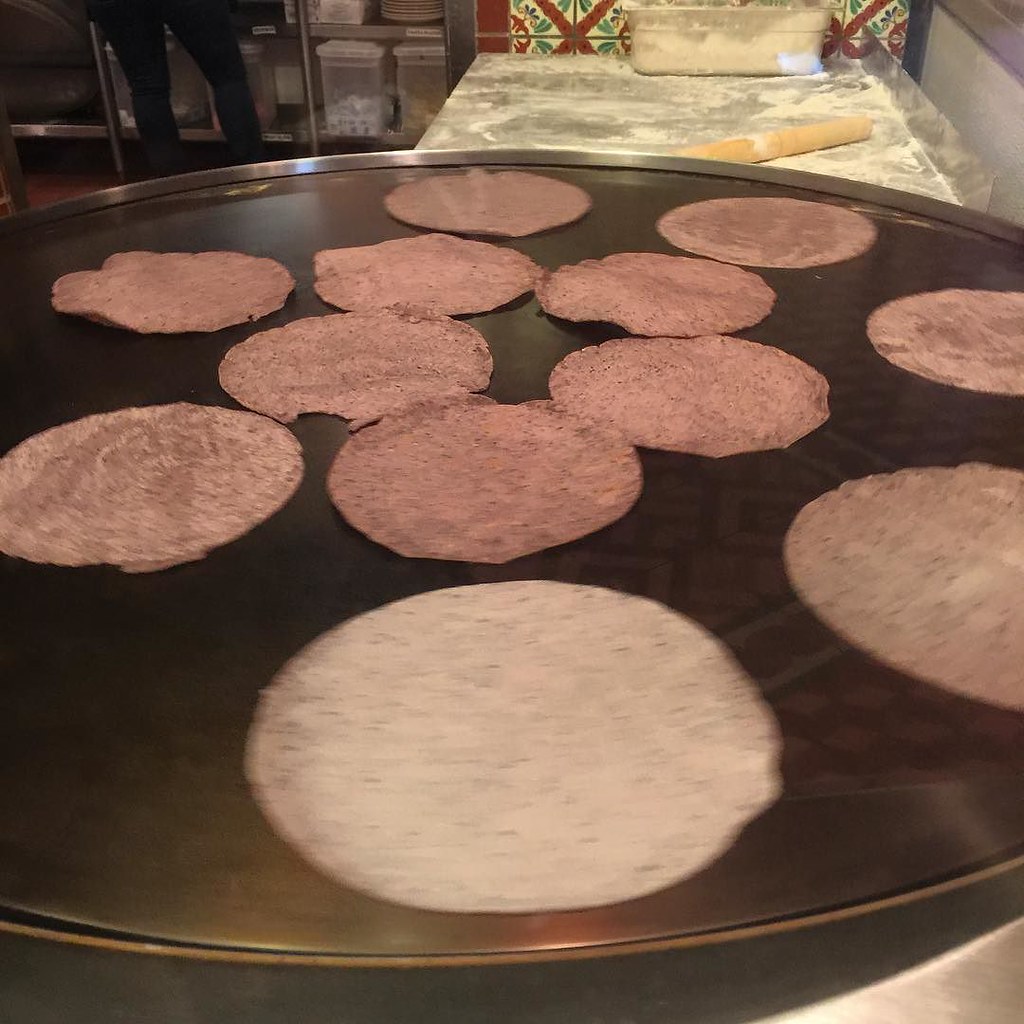In this color photograph taken in a kitchen, a large circular grill occupies 85% of the frame, with several pita breads arranged for cooking. The pitas, browned on one side, await turning, with one in the blurred foreground showcasing bubbles forming on its surface. Above the grill, a stainless steel worktop holds a large rolling pin and a plastic container of flour. Nearby, a marble countertop in gray and cream hues features a dark red backsplash with green leafy patterns. A person dressed in black slacks stands on the left, near shelves holding plastic containers. In the background, parts of an oven, a refrigerator, and storage bins are visible, contributing to the organized yet busy ambiance of the kitchen.